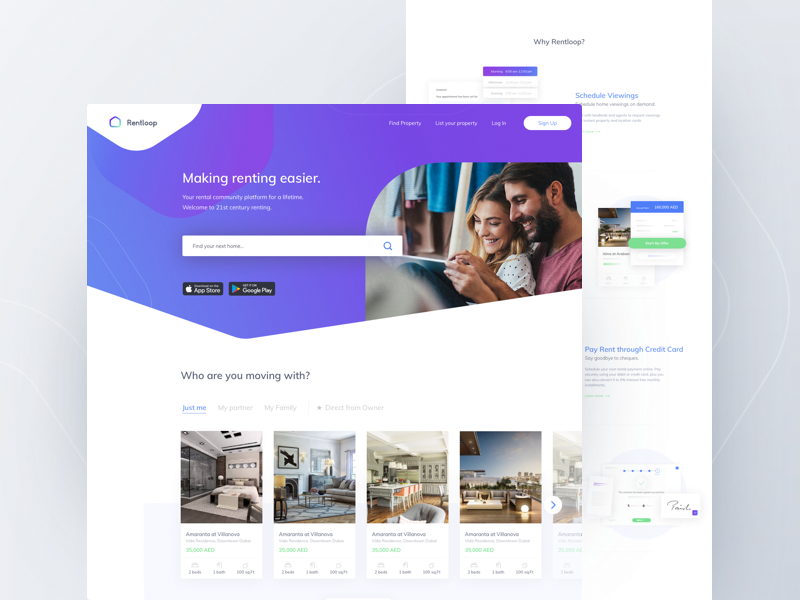**Detailed Caption:**

The screenshot depicts a user interface from Rentloop, though it appears to be a standalone application rather than a webpage, given the absence of typical browser elements. The main background window showcases a section titled "Why Rentloop?" with various subheadings such as "Schedule Viewings" and "Pay Rent Through Credit Card," though the low resolution renders most text unreadable. This content is presented in a vertical white ribbon aligned to the right side of the window, accompanied by a mix of text and graphics.

Overlaying this primary window is another Rentloop interface, prominently displaying the slogans "Making Renting Easier" and "Your Rental Community Platform for a Lifetime. Welcome to 21st Century Renting." At the top, navigation tabs offer options such as "Find Property," "List Your Property," "Log In," and "Sign Up." A cheerful image of a man and woman laughing while looking at a tablet reinforces the platform's user-friendly vibe. The color scheme prominently features purple, blue, and green hues. Below this overlay, there's a side-scrolling gallery featuring various images of bedrooms, houses, and rooms, captioned with questions like "Who are you moving with?" This secondary window emphasizes Rentloop's focus on facilitating moving and renting experiences.